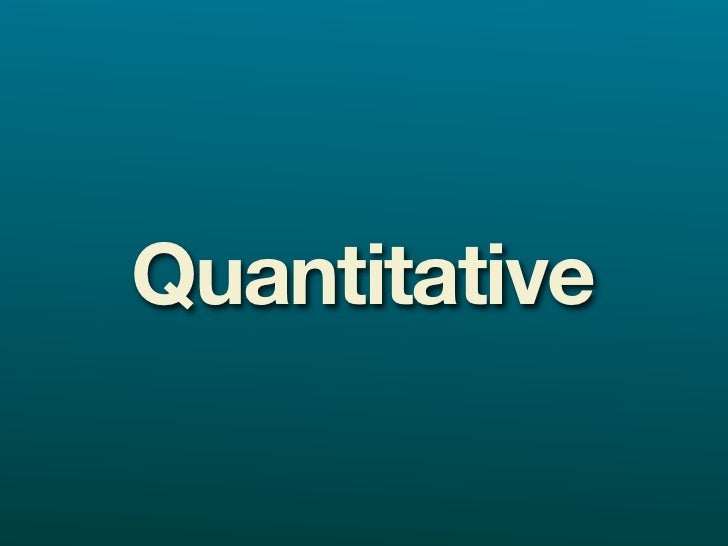The image features a rectangular, computer-generated background that transitions smoothly from a light teal at the top to a darker teal at the bottom. Measuring approximately 8 inches wide by 6 inches tall, the simplicity of its design makes it ideal for use in a presentation. Centered on this gradient backdrop is the word "Quantitative," written in white Times New Roman font with a capital "Q" followed by lowercase letters. The text is accentuated by a subtle dark gray shadow effect that adds depth. There are no other elements present in the image, emphasizing its clean and straightforward aesthetic.